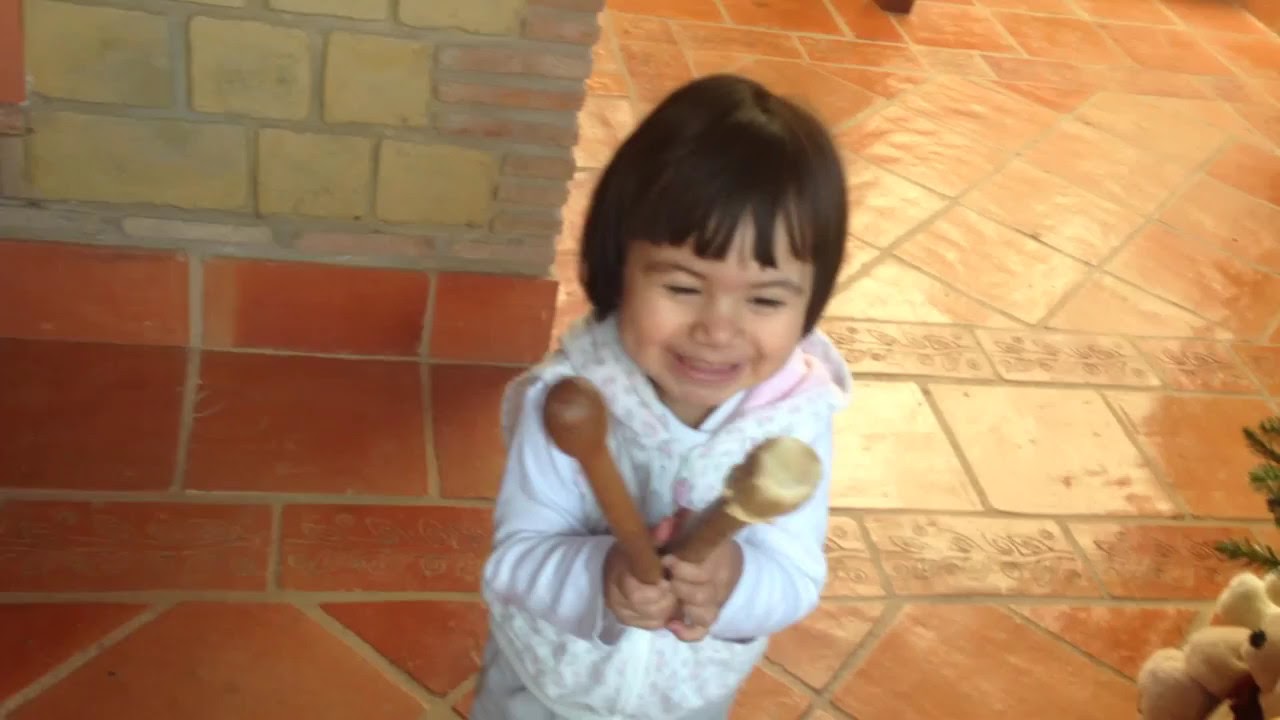The photograph depicts a joyous toddler, approximately one to two years old, standing inside what appears to be a well-lit building with horned tiles on the floor and a brick wall in the background. The toddler, who might be of Asian or Latin American descent, has short black hair and a radiant smile on her light-skinned face as she energetically holds two large wooden drumsticks. She is dressed in a white hooded sweater adorned with delicate pink flowers and complemented by grey sweatpants. The setting, potentially a store or a commercial space, showcases a red and beige tiled floor with some tiles engraved with floral patterns. In the bottom right corner, there are visible pine branches from a small potted plant and parts of what appear to be two teddy bears, one partially cropped out. The overall scene exudes warmth and brightness, captured with high clarity.